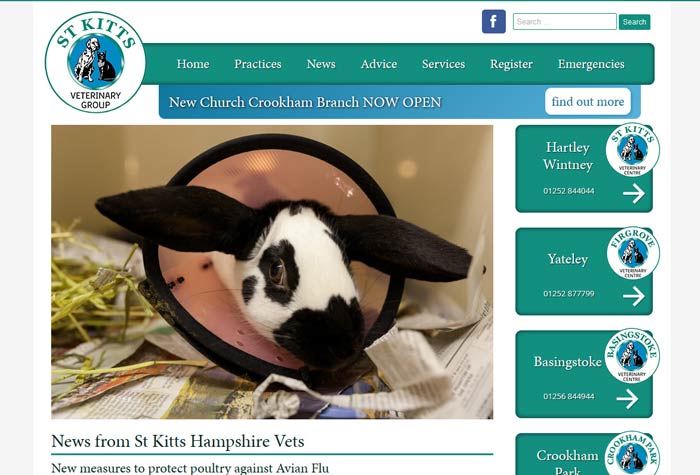The website page predominantly features animal-friendly content and showcases the majority of its layout. Centrally placed, there is an image of a rabbit wearing a protective neck device, featuring a pinkish hue with black borders and equipped with a few holes. The rabbit's ears, black and flopping sideways, add to its endearing appearance. One visible eye has a brown pupil set against the predominantly white fur of its face, complementing the brown area around its nose.

At the top of the page, the title "ST Kitts Veterinary Group" is prominently displayed. The navigation menu, situated within a light green bar, includes options such as Home, Practices, News, Advice, Services, Register, and Emergencies. Above this menu, there's a Facebook icon and a search field with a corresponding search button.

Below the menu bar, a light blue section announces the opening of the "New Church Cookham Branch," accompanied by a "Find Out More" link. Following this section, the names of various locations—Hartley, Whitney, Gatley, Basingston, Stoke, and Crookham—are listed, each with corresponding symbols and right-pointing arrows for further navigation.